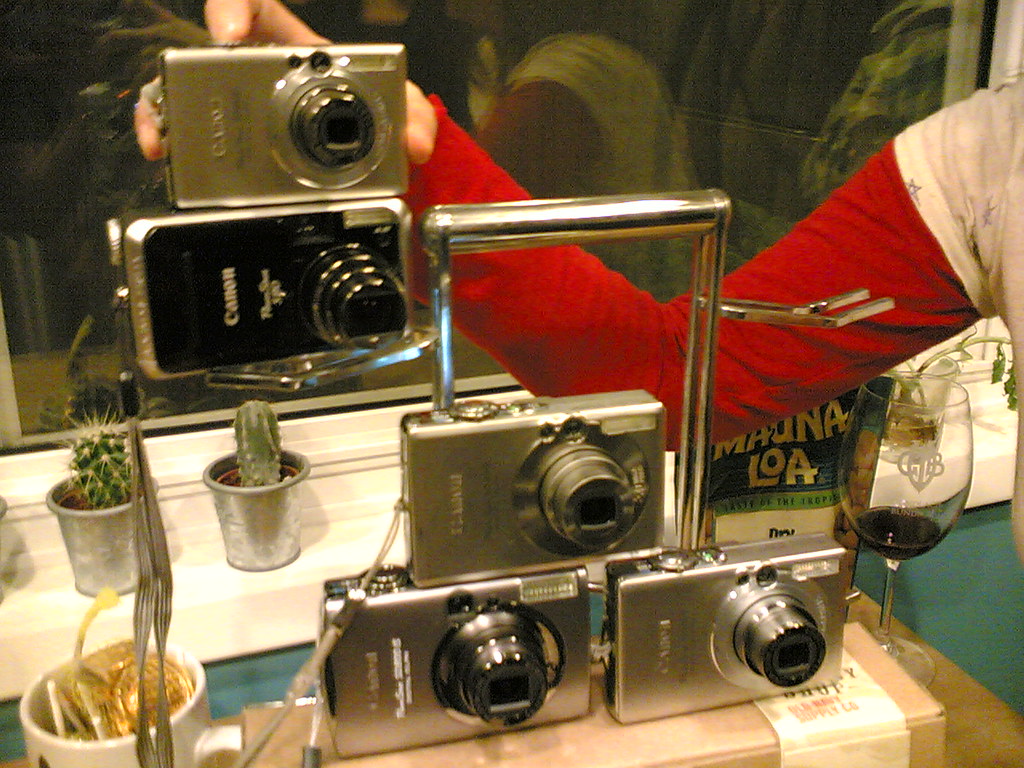The colour photograph captures a detailed scene within what appears to be a personal home. At the center, a collection of five compact digital cameras is meticulously arranged on what seems to be a silver stand or shelf. Each camera's lens is prominently extended, pointing directly at the viewer. Four of the cameras exhibit shades of silver, while one stands out in black. The brand Canon is clearly visible on at least two of the cameras, although the image is slightly soft in focus, rendering other written details indistinct.

To the left side of the display, a person's arm, clad in a long-sleeved red T-shirt beneath a white short-sleeved T-shirt, reaches into the frame, hand grasping a silver Casio camera. Below this Casio, a black Canon camera hangs, its handle discernible. Further to the left under the person's arm, a wine glass containing a small amount of red wine and a bag labeled "Mauna Loa" can be seen. 

The cameras are flanked by small potted cacti in silver pots on a white windowsill. Behind this arrangement, a large window provides a reflective backdrop, faintly mirroring the scene and adding depth. Additionally, a cup filled with miscellaneous items sits on the left side of the camera stack, completing the eclectic, homey setting.